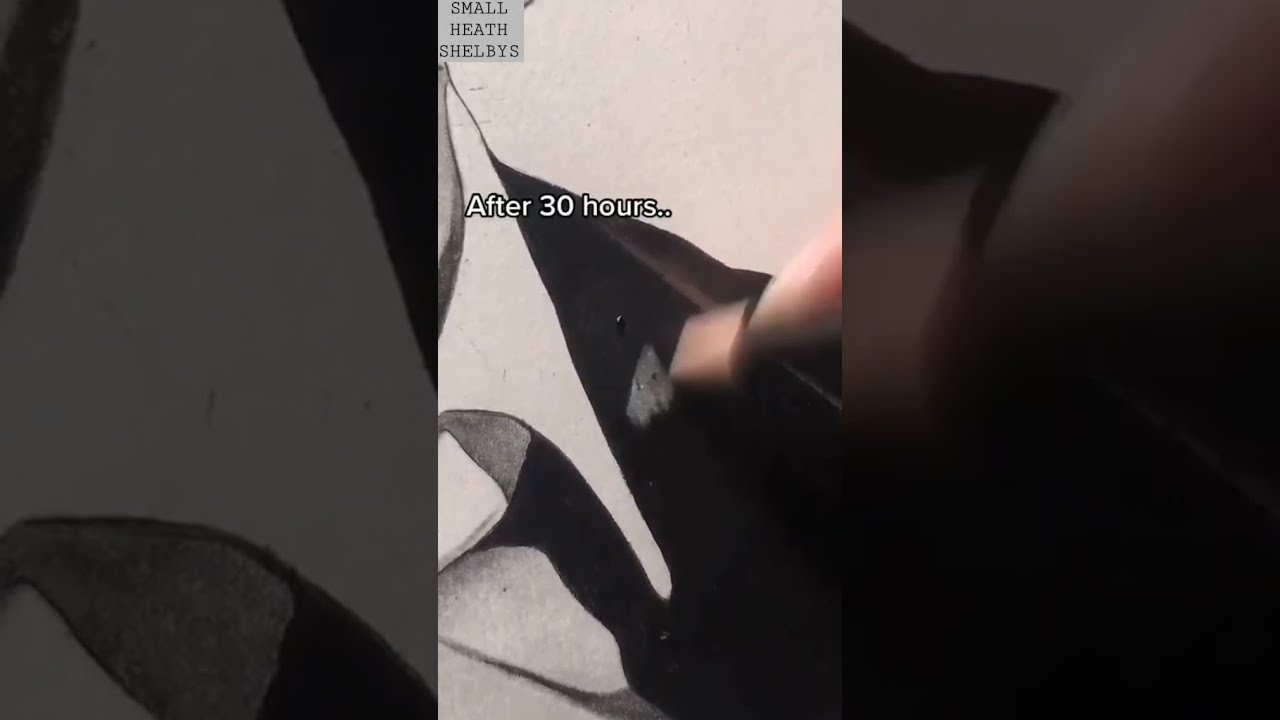The image appears to be a blurry, zoomed-in photograph or possibly a screenshot of artwork in progress, divided equally into three sections. The left section is dark and unclear, featuring faint elements of the artwork. The middle section is lighter and more distinguishable, showing what might be a hand or brush working on the piece. This section contains white text stating "after 30 hours..." Below this is a small gray box with the black text “Small Heath Shelby's.” The right section includes an unclear tan object, possibly part of a leg or foot. Overall, the image displays shades of gray, black, white, and off-white, and might have originated from a mobile application interface or video.